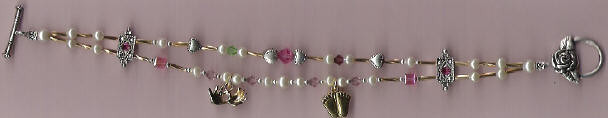The photograph showcases a beautifully intricate necklace spread out in a line across a dark brown or peach-colored surface. This exquisite piece of jewelry prominently features layers of lustrous white pearls interspersed with elegant gold spacers, creating an alternating pattern of pearls and gold. In addition to the pearls, the necklace is adorned with a variety of gemstones and charms, including a winged floral design on the far right end and a small scroll-like charm on the far left. Scattered along the length of the necklace, there are also red beads and pink rhinestone-like accessories, adding a touch of vibrant color and sparkle. Midway across, a small metallic symbol is attached to two white beads, complementing the overall opulence of the design. The ends of the necklace feature silver tips, with one end forming a round loop, enhancing its classy and sophisticated look.